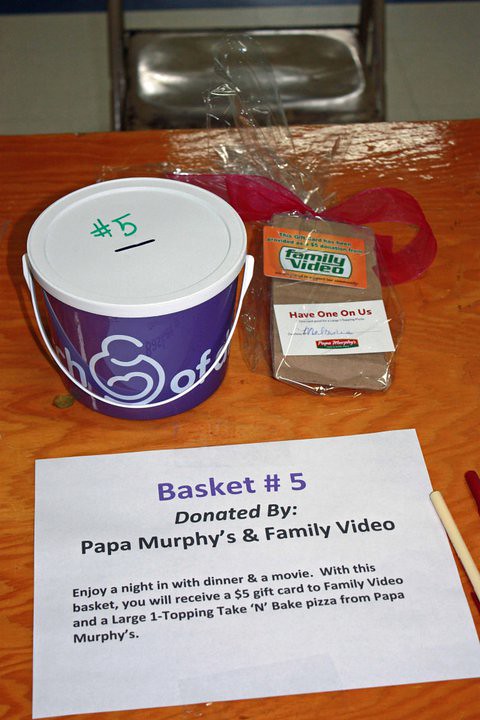On a wood-grained table sits a metal bucket emblazoned with the March of Dimes logo, featuring a removable lid with a slot cut out for coins or tickets and marked with the number five in green marker. To the right of the bucket, there is a cellophane-wrapped brown paper bag with an orange tag reading "Family Video" and "Have one on us," hinting at a giveaway item, possibly a VHS tape or a movie. Beneath the bucket, a piece of printer paper in purple declares "Basket Number Five," and in black text, it states, "Donated by Papa Murphy's and Family Video." The paper further explains, "Enjoy a night with dinner and a movie. With this basket, you'll receive a $5 gift card to Family Video and a large one-topping take-and-bake pizza from Papa Murphy's." The entire setup appears to be a raffle prize or a charitable giveaway aimed at offering an enjoyable evening with a movie and a meal.